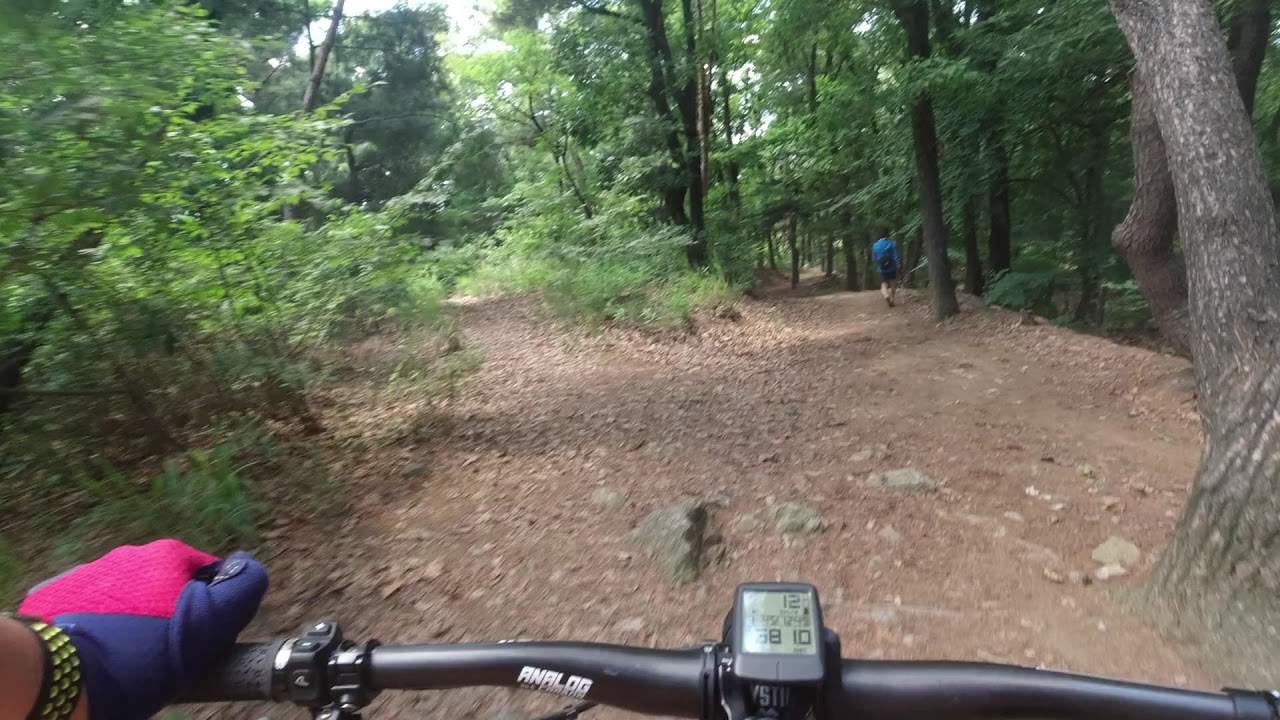This photograph, presumably taken from a GoPro, captures the point of view of someone riding a mountain bike on a dirt trail through a wooded area. The central focus is on the black or dark gray handlebars, which feature a digital speedometer displaying numbers, and a white logo on the left side reading "Analog." The rider's left hand, clad in a glove that is a blend of pink, blue, and possibly yellow, is visible on the handlebar. The rider also sports a black-and-yellow sports bracelet. The dirt trail, brown in color, winds through dense greenery, with trees lining both sides. Ahead, a person wearing a long-sleeved blue shirt, shorts, and carrying a knapsack on the right shoulder walks along the same path. The overall scene is set during daytime, under the canopy of trees with patches of sunlight filtering through the leaves.